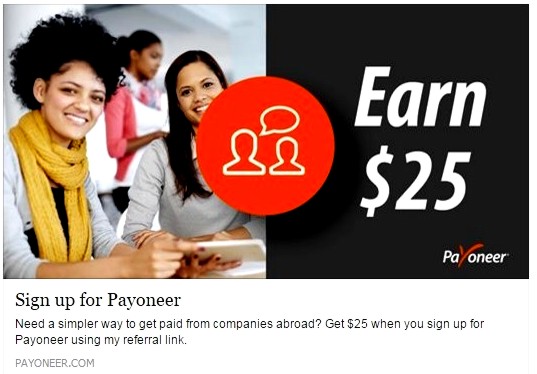This advertisement for Payoneer is split into two distinct halves within a wide rectangular layout. The left half features an image of three women: the foreground shows two women with dark complexions and gray shirts, one with an afro and a yellow-gold scarf, and the other with long hair. In the background, a third woman, wearing a pink shirt with her hair tied in a ponytail, is slightly obscured. There's a prominent red circle overlapping both halves, containing white outlines of two people with a speech bubble between them.

The right half of the ad has a solid black background with white text, featuring the capitalized phrase "EARN $25." In the bottom right corner, "Payoneer" is displayed, highlighted by a large red 'Y' in the word. Below the imagery, the text reads: "Sign up for Payoneer. Need a simpler way to get paid from companies abroad? Get $25 when you sign up for Payoneer using my referral link." The company's website, "www.payoneer.com," is written in light gray font beneath the call-to-action.